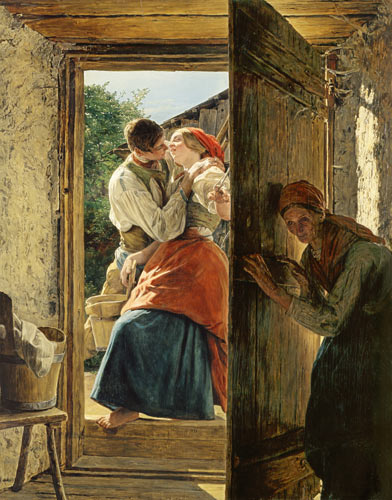This detailed painting depicts a rustic scene set in an old stone house. In the center, an open wooden door frames a tender moment between a man and a woman, seemingly on the verge of a kiss. The man, standing to the left, has brown hair and wears period-appropriate attire. He supports the woman who appears faint, possibly swooning, dressed in an orange apron and a long blue dress with a red headscarf. To the right, an older woman, partially hidden behind the door, watches attentively, perhaps eavesdropping, dressed in a brown headband and a long blue dress.

Inside the home, visible to the bottom left of the image, a small stool holds a washbasin with a tan bucket and a white cloth, adding to the domestic atmosphere. The interior features walls on both sides and a dark brown ceiling, evoking a warm, lived-in feel. Through the doorway, in the distance, a tree is visible, indicating an outdoor setting beyond the house and capturing a slice of sky, suggesting it is daytime.

The painting’s color palette is rich and varied, featuring earth tones like brown and tan, along with vibrant touches of blue, orange, green, and red. The image is evocative of a bygone era, its painterly style providing a sense of timelessness, making it an artifact likely to be admired in a museum.